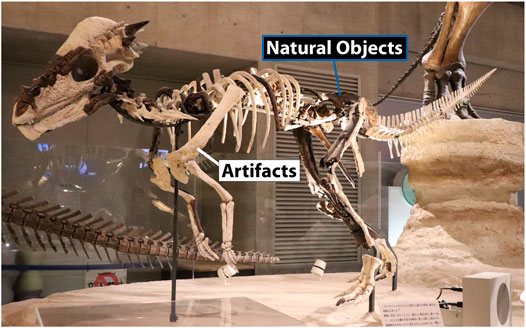The photograph, taken inside a museum, features a partial assembly of what appears to be a smaller dinosaur skeleton, possibly a Velociraptor. The skeleton is displayed prominently on a polished marble base. Composed of both dark-colored, genuine fossils and light-colored, human-made replicas, the display illustrates the completion of the skeletal structure. The dinosaur, characterized by a larger head with horns and four similarly-sized legs, is labeled with annotations clarifying the distinction between natural objects and artifacts. In the background, one can identify the tail of another dinosaur and the foot of a much larger specimen, also part of the exhibit. The scene is set against the museum's stone walls, interspersed with vents and additional glass-covered exhibits.